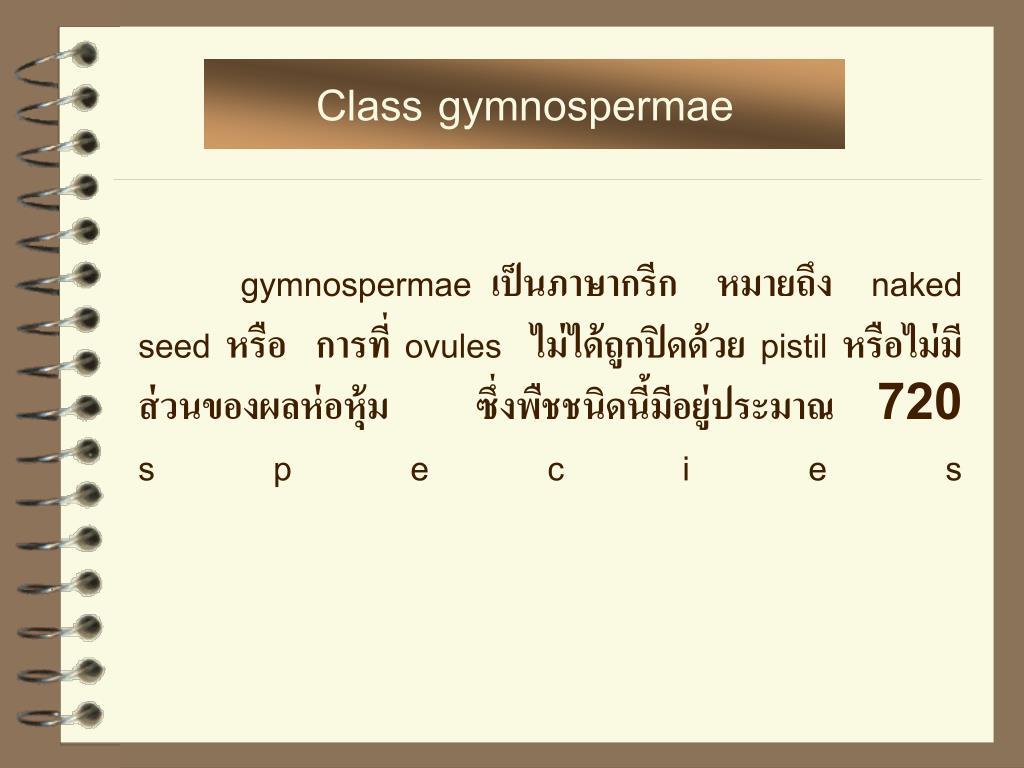The image depicts a stylized illustration of a spiral-bound notebook resting on a golden surface. The metal spiral binding on the left is silver, and the page itself is pale yellow with a shaded gray and brown title box at the top. The title "Class Gymnospermae" is prominently displayed, spelled out as G-Y-M-N-O-S-P-E-R-M-A-E in beige text against the brown background. Below the title is a thin gray line, followed by a mixture of English and a non-Roman script. The text sequence in English includes the words: "Gymnospermae," "naked," "Seed," "Ovules," "Pistil," and "Species," interspersed with characters from the foreign language. Also, there is the number "720" in large block capitals before the final word "Species," which is spelled S-P-E-C-I-E-S with evenly spread letters. The entire background of the image is light brown.